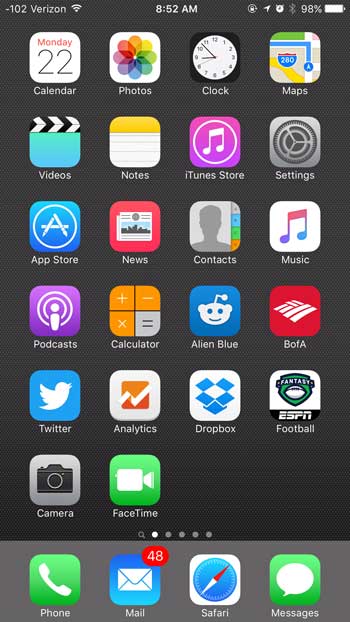This image is a detailed screenshot of an individual's smartphone home screen, displaying a variety of app icons on a black background. At the very top of the screen, the status bar indicates a signal strength of -102 dBm on Verizon's network, with active Wi-Fi connectivity. The current time is displayed as 8:52 AM, and several status icons are visible to the right, including a locked circle, a location services arrow, an alarm icon, Bluetooth connectivity, and a battery level at 98%.

The layout of the home screen features app icons arranged in a grid of four columns across and seven rows down. Starting from the top left, moving left to right, the first row includes the Calendar, Photos, Clock, and Maps apps. The second row features Video, Notes, iTunes Store, and Settings. The third row contains the App Store, News, Contacts, and Music apps. In the fourth row, we see Podcasts, Calculator, Alien Blue, and B of A (Bank of America). The fifth row displays icons for Twitter, Analytics, Dropbox, and ESPN Football. In the sixth row, there are just two apps: Camera and FaceTime.

Beneath these app icons, there is a series of five dots indicating that this is the first of five possible home screen pages. At the bottom of the screen, in a lighter gray dock, are four essential apps: Phone, Mail (which shows 48 unread emails), Safari, and Messages.